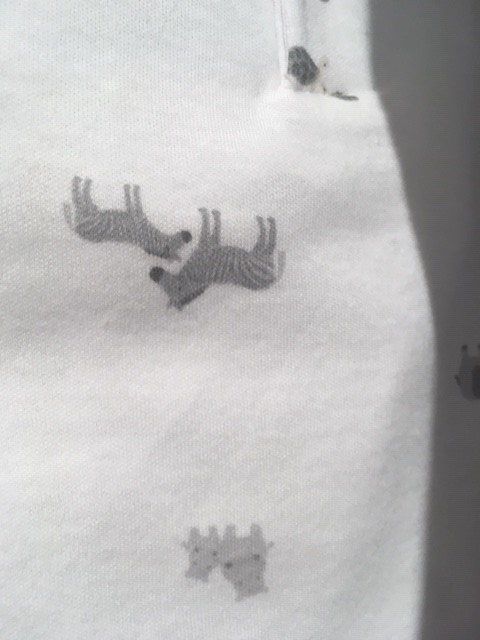This is a black-and-white photograph of a piece of clothing, likely a blanket or a garment, that is taller rather than wider by approximately 50%. The fabric has a faint grid pattern and features multiple wrinkles and folds, emphasizing its textured and draped nature. The lighting accentuates the monochromatic tones, revealing various design elements on the fabric. There are two upside-down zebras that are grey and white with one slightly larger than the other, intersecting by their heads and facing each other. These are located midway up the image. At the bottom center of the fabric, two giraffe heads, also in shades of grey, look directly towards the viewer. A shadow encroaches on the right side of the picture, suggesting the presence of additional, albeit obscured, designs. Towards the top of the image near the center, there's a small dark circle resembling a folded cloth, likely indicating the opening of the garment.